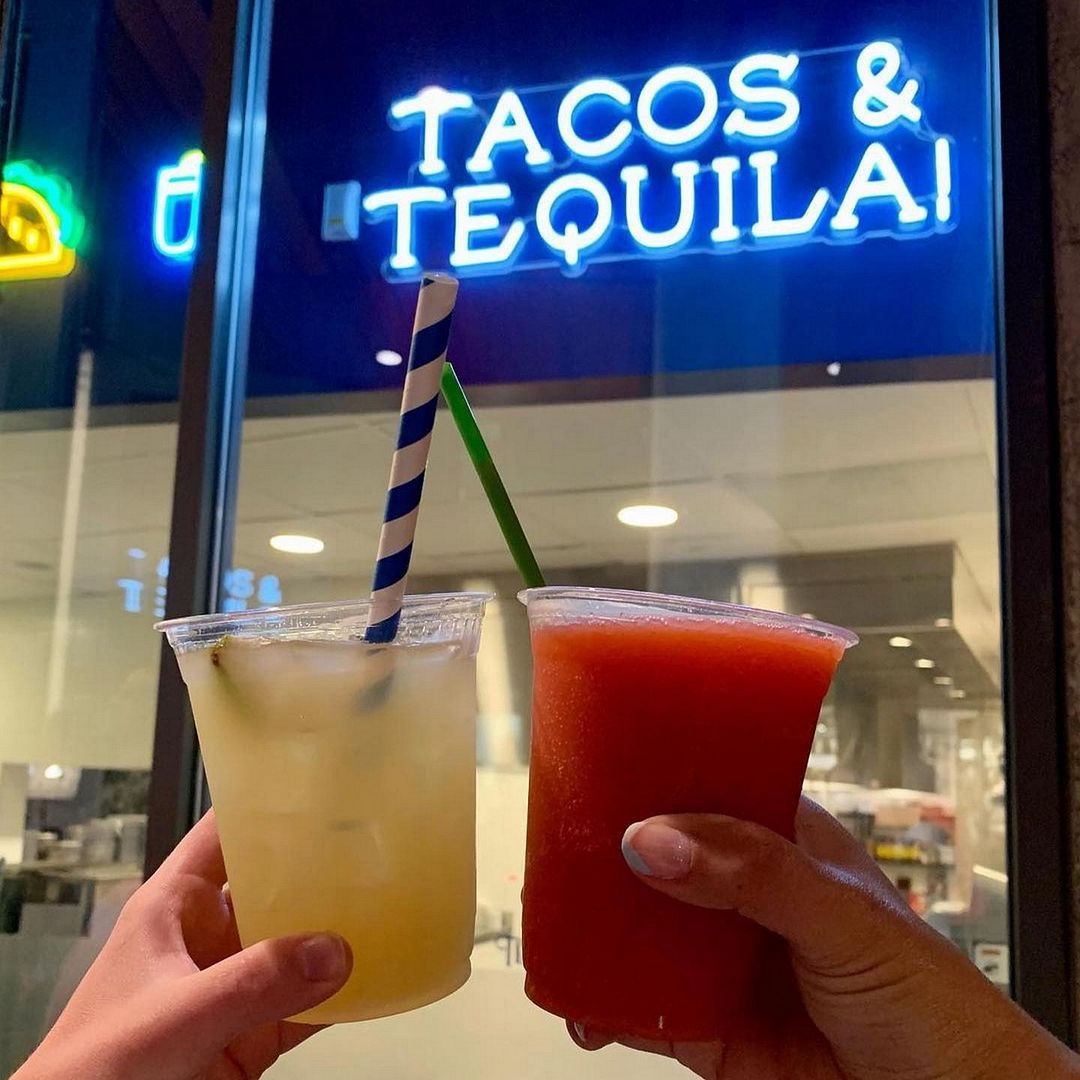The vibrant nighttime photograph captures two hands holding drinks in a celebratory gesture in front of a restaurant window. The left hand, possibly belonging to a Caucasian female, clutches a clear glass filled with a light yellow drink, adorned with a prominent white and blue striped straw. The right hand, larger with a long thumbnail, holds a red slushy drink through a green straw, likely belonging to an individual of Spanish or African-American descent. Behind the hands, the image reveals the restaurant's stylish interior, characterized by its white ceiling with two circular white spotlights and a blue ceiling section above. Visible through the clear glass windows with vertical black metal bars, a lit neon sign proclaims "Tacos and Tequila," alongside an illustrated taco and drink, enhancing the lively, festive atmosphere of the scene.